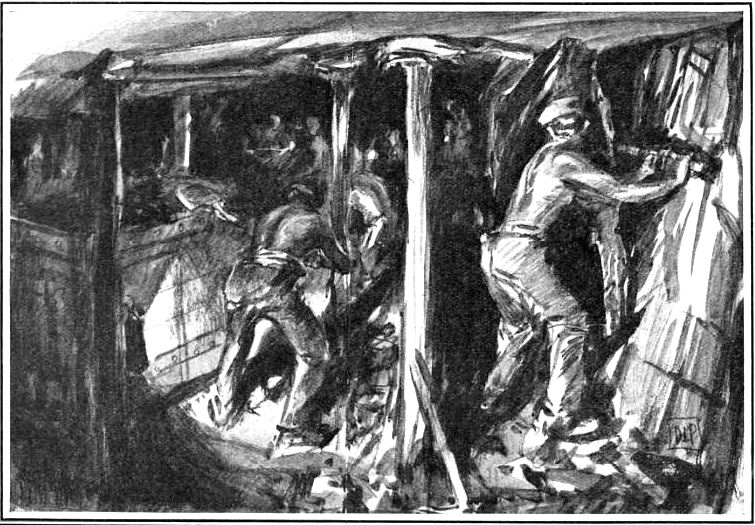The image is a highly detailed, black-and-white charcoal drawing of shirtless men working in a narrow, cramped, and dark underground space. Most of the men, who appear to be miners, are positioned with their backs toward the viewer and are engaged in various tasks such as digging into the walls and shoveling material into a boxy mine cart, which is secured to a rail system and features bolts on its sides. The single source of light in the scene is a lantern hanging from a support beam on the left side, casting limited illumination across the dim, oppressive environment.

Prominently on the right-hand side of the image, a muscular man, bent over and wearing pants and a hat, is pushing against a wall, possibly trying to brace it as if it might collapse. Next to him, another similarly dressed man is also pushing against a wall, reinforcing the notion that they may be trying to prevent structural failure within the mine. The background features additional figures of men, drawn as smaller outlines to suggest distance.

The composition is rich with intricate details, emphasizing the intensity and exertion of the miners' labor. At the bottom right corner of the drawing, the artist has signed their work with the initials "D.I.P." enclosed within a black-bordered square.